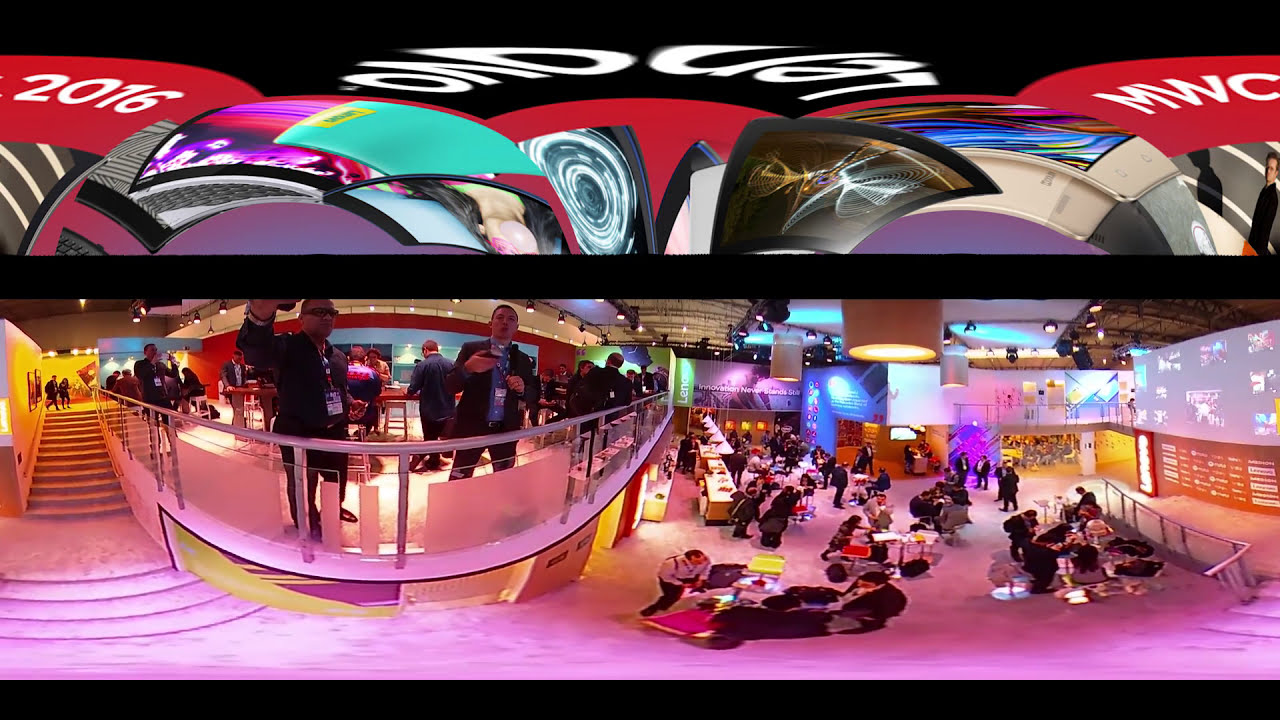The vertical rectangular image, taken with an unusual lens, depicts a vividly colored indoor setting that seems to straddle between a convention hall and a club-like environment. It has a distinctive thin black edge at the top and bottom. Dominating the lower two-thirds, there is a pink stairway on the left leading to an upper area where people stand and overlook the scene below, suggesting an interactive or observatory space. Beneath this balcony, the floor area is bustling with individuals either standing, sitting at tables, or congregating, with many of them wearing badges, hinting at a possible convention or conference. The lighting is dynamic, casting a pink reflection on the ground and featuring various hues like blue, yellow, green, purple, and more. The setting includes several screens in the background, further enhancing the vibrant atmosphere. In the upper portion of the image, there appears to be a design resembling race cars, adorned with multiple colors and prominently displaying the text "2016 MWC" in red, possibly indicating the event or brand logo, linking it to a convention theme. The overall setting is richly colored with pink, purple, yellow, gold, silver, blue, green, orange, teal, black, and gray scattered throughout the image, contributing to its energetic and multifaceted character.